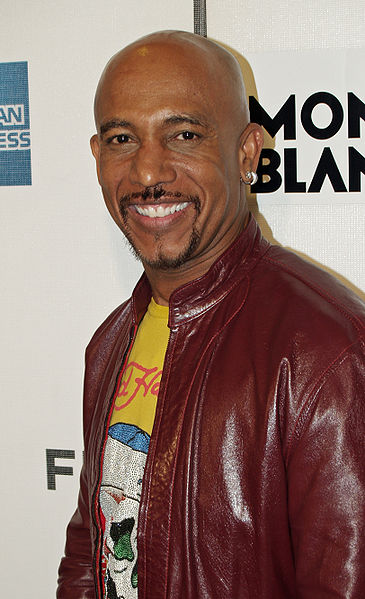The photograph features Montel Williams, a notable African-American talk show host, standing against a backdrop adorned with logos from Mont Blanc and American Express, hinting at a promotional or sponsored event. Montel is smiling and has a bald head, with a neatly groomed black mustache and goatee. He sports a distinctive look with silver earrings in his left ear. He is dressed in a maroon leather jacket over a mustard yellow Ed Hardy t-shirt. The t-shirt displays a vividly intricate graphic design embellished with beading, sequins, and colors like white, blue, green, and hints of red. Despite the vibrant detailing, the exact design of the t-shirt remains unclear due to the jacket partially obscuring it.